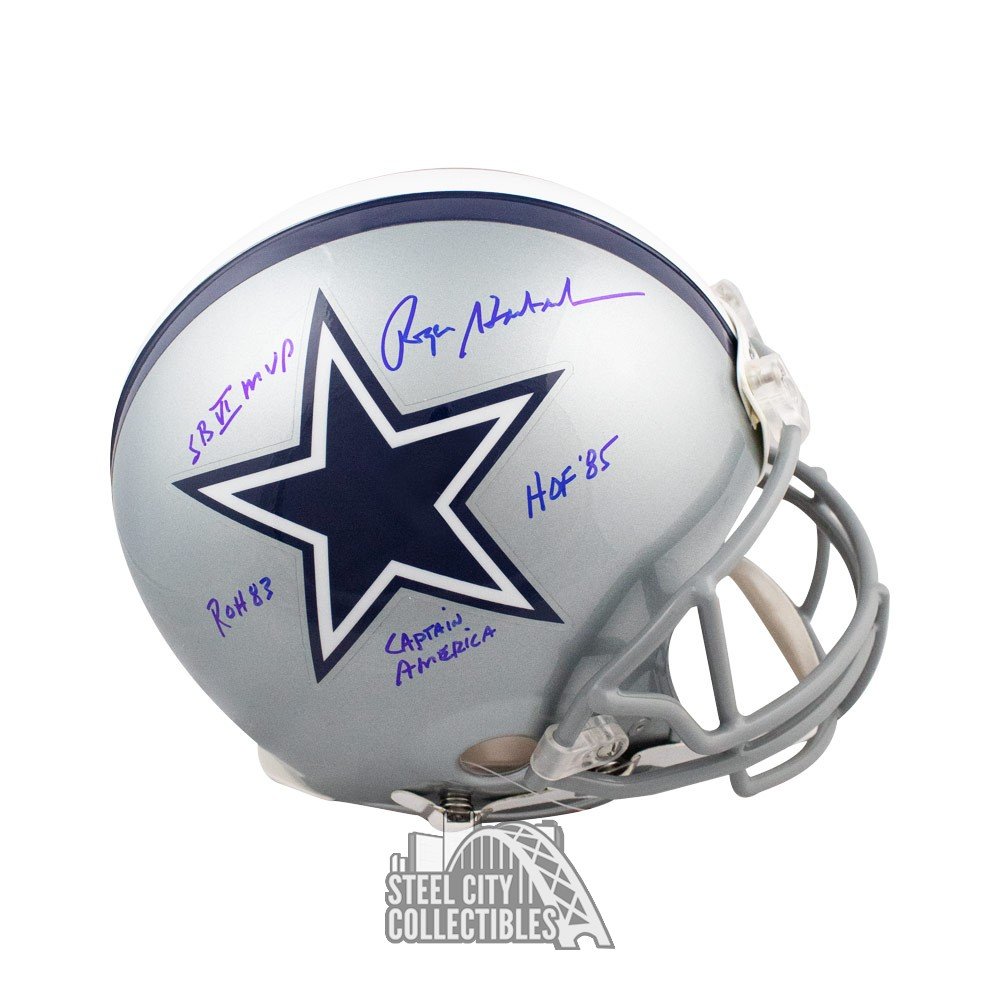This image depicts a Dallas Cowboys football helmet, detailed with a combination of signatures and notable inscriptions. The helmet features the iconic blue star logo with both white and dark borders, set against a silver-gray background with a blue stripe running across the top. The helmet includes a gray faceguard and a translucent clip on the side, which seems somewhat flimsy, suggesting that this could be a toy-scale replica rather than a full-size, game-used helmet.

The helmet is adorned with various inscriptions in blue marker, prominently featuring "SB6 MVP" and the nickname "Captain America." Additionally, "ROH 83" and "HOF 85" are also inscribed, indicating significant accolades. A notable cursive signature is displayed beneath the star logo, and despite its stylized nature, it contributes to the item's uniqueness.

Additionally, located at the bottom of the helmet is a small emblem that reads "Steel City Collectibles" in white text on a gray background. The entire backdrop of the image is stark white, giving the impression that the helmet is placed in isolation.